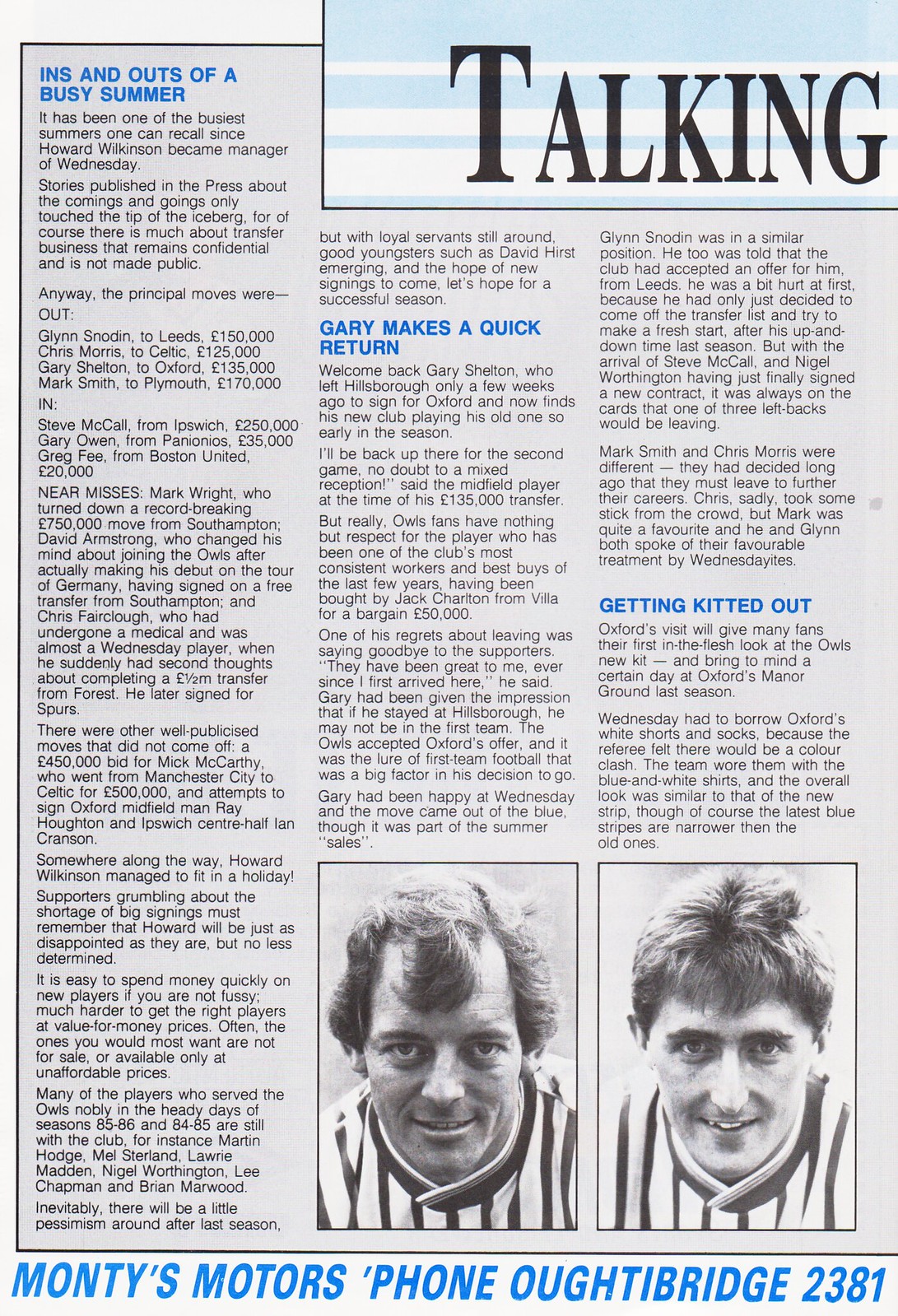The image depicts a black and white newspaper or magazine snippet with elements of blue text. At the very top, there’s a banner featuring the word "TALKING" in large black letters. Following that, there’s a lengthy article in black text accompanied by several blue headlines. The first headline reads "Ins and Outs of a Busy Summer," positioned at the upper left and partially extending into the middle column. The middle column features the headline "Gary Makes a Quick Return," and the third column is titled "Getting Kitted Out." Each section appears to present separate articles, with the third article likely continuing onto another page that isn't visible in the image. At the bottom of the page, there's blue text that reads, "Monty's Motors, phone Outerbridge 2381." Additionally, the bottom of the page features two black and white photos of adult males. Both men have short light brown hair and are smiling, dressed in vertically striped dark and white outfits.